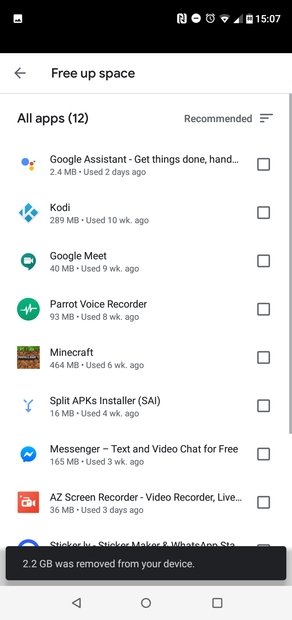### Caption:

The image showcases a screenshot of a mobile device's screen displaying a list of apps. At the very top of the screen, there is a black status bar featuring white icons, including a clock (showing the time, 15.07), Wi-Fi signal, battery level, and other circular icons.

Underneath the status bar, a white rectangular header reads "Free up space" in black text, accompanied by a left-facing arrow on the left, which likely serves as a back button. A thin gray line separates this header from the main content below.

The main content begins with a horizontal layout: on the left, "All apps (12)" is displayed, indicating there are 12 apps listed; on the right, in dark gray text, it reads "Recommended" followed by an icon resembling a menu with three horizontal lines of varying lengths.

Below this section, a list of apps is displayed:
1. **Google Assistant** - Icon: Blue circle with a yellow object
   - Info: 2.4 MB, used two days ago
   - Checkbox: Empty

2. **Kodi** - Icon: Diamond-shaped logo made of blue squares
   - Info: 289 MB, used 10 weeks ago
   - Checkbox: Empty

3. **Google Meet** - Icon: Greenish-blue speech bubble with a camcorder icon
   - Info: 40 MB, used nine weeks ago
   - Checkbox: Empty

4. **Parrot Voice Recorder** - Icon: Green circle with white voice recording lines
   - Info: 93 MB, used eight weeks ago
   - Checkbox: Empty

5. **Minecraft** - Icon: Minecraft game image with land and green grass
   - Info: 464 MB, used six weeks ago
   - Checkbox: Empty

6. **Split APKs Installer (FAI)** - Icon: Light blue downward-facing arrow
   - Info: 16 MB, used four weeks ago
   - Checkbox: Empty

7. **Messenger - Text and Video Chat for Free** - Icon: Blue chat bubble with a white lightning sign
   - Info: 155 MB, used three weeks ago
   - Checkbox: Empty

8. **AZ Screen Recorder - Video Recorder, Live...** - Icon: Reddish-orange square with a white camcorder
   - Info: 36 MB, used three days ago
   - Checkbox: Empty

9. **Stickerly Sticker Maker and WhatsApp...** - Partially visible icon: Blue circle
   - Info: Mostly covered by a notification box

At the bottom of the screen, a black notification box states "2.2 GB was removed from your device" in gray font. Below this notification, the navigation bar features a left-facing triangle back button, a circle home button, and a square overview button.